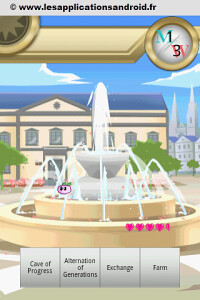Caption: 

This screenshot appears to be from an old computer game, possibly in French, as suggested by the website URL "lessapplicationsandroid.fr" displayed at the top. Despite the French URL, the text within the game is in English. The scene depicted presents a large, stately mansion in the background, featuring a grand, three-tiered circular fountain in the foreground with water gracefully cascading from each level. The game's interface shows the player character possessing four and a half hearts, indicating their current health status. Additionally, a grey menu box overlays the scene with the options: "Cave of Progress," "Something of Generations," "Exchange," and "Farm," likely representing different gameplay areas or missions. At the top of the screen, a gold bar with a gold star is also visible, serving as an in-game image or icon.